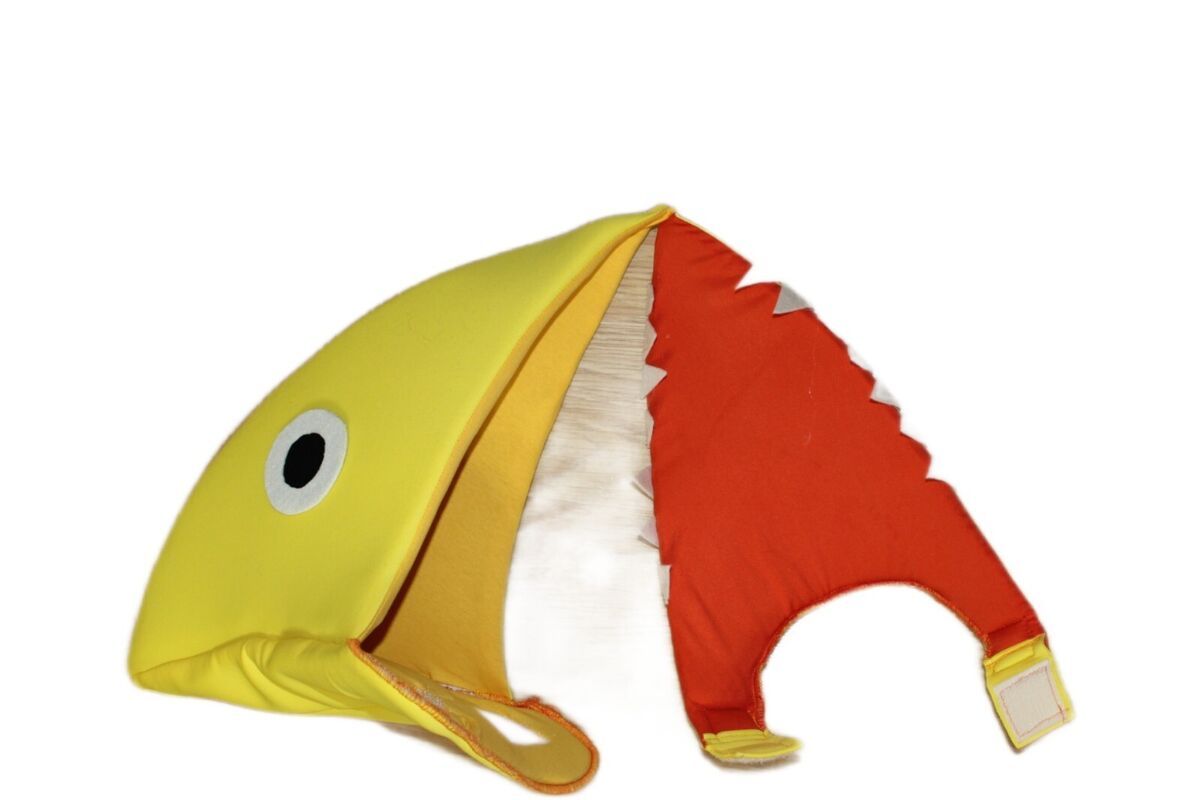This full-color photograph presents a peculiar, vividly colored, and seemingly sewn object against a white background, providing no additional context or text. The object, speculated to be either a hat or a mask, features a yellow, triangular section on the far left side, adorned with a white circular "eye" bearing a black pupil. Beneath this "eye" is a line suggesting a mouth. Moving rightwards from the yellow section, there is a darker, almost gold-yellow part followed by a white segment. The rightmost part of the object is red, extending down into two points at the bottom right corner, both equipped with white Velcro patches. These Velcro patches imply that the object can be fastened, potentially to itself or another item. The puzzling design suggests it could be an imaginative headpiece or mask, perhaps resembling a bird or fish, most likely intended for a child.